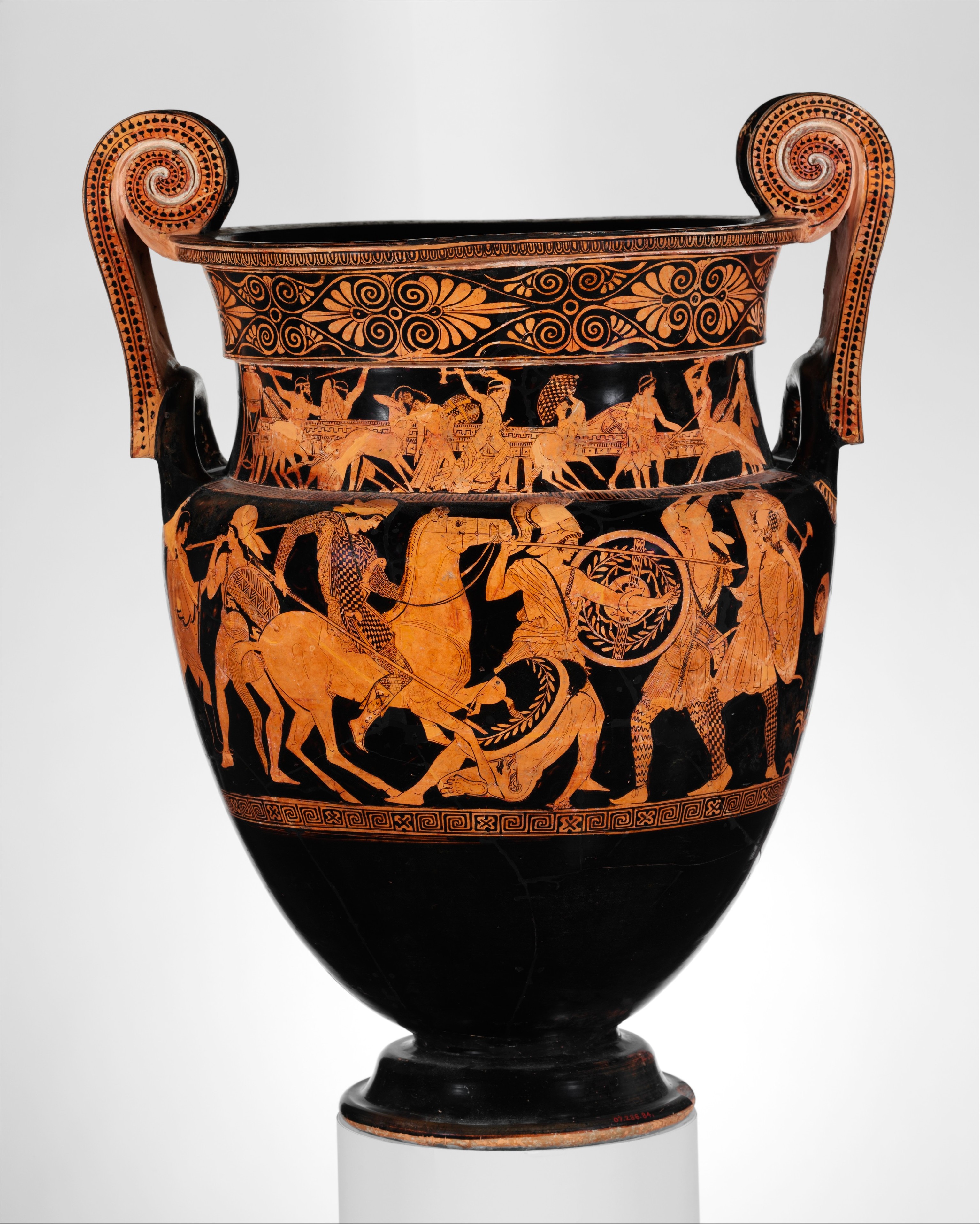This image portrays a classical Grecian urn, meticulously displayed on a tailored white pedestal that accentuates its elegant form, suggestive of a museum exhibit. The urn itself is an exquisite black glazed ceramic piece, distinguished by its two upward-curving handles, adorned with inscribed black dots. These handles elegantly frame the urn's mouth, leading the eye to a decorative rim featuring intricate curlicues and stylized floral or leaf patterns in a reddish-golden hue.

The body of the urn is primarily black, providing a striking contrast to the detailed scenes depicted upon it. The main decorative band, broad and encircling the middle of the urn, vividly portrays a chaotic battle scene with warriors both on horseback and on foot, wielding spears and shields. The riders are equipped with classical Trojan-style helmets and round shields, emphasizing the Grecian theme. 

Beneath this prominent battle depiction, a narrower strip continues the narrative with additional figures possibly in combat, though the details are finely rendered and somewhat diminutive. The figures throughout are painted in a burnt orange-red color, enhancing the dramatic visuals against the dark ceramic backdrop. 

Overall, this urn is a magnificent example of classical artistry, combining elegant form with intricate storytelling through its detailed and vivid warrior scenes.